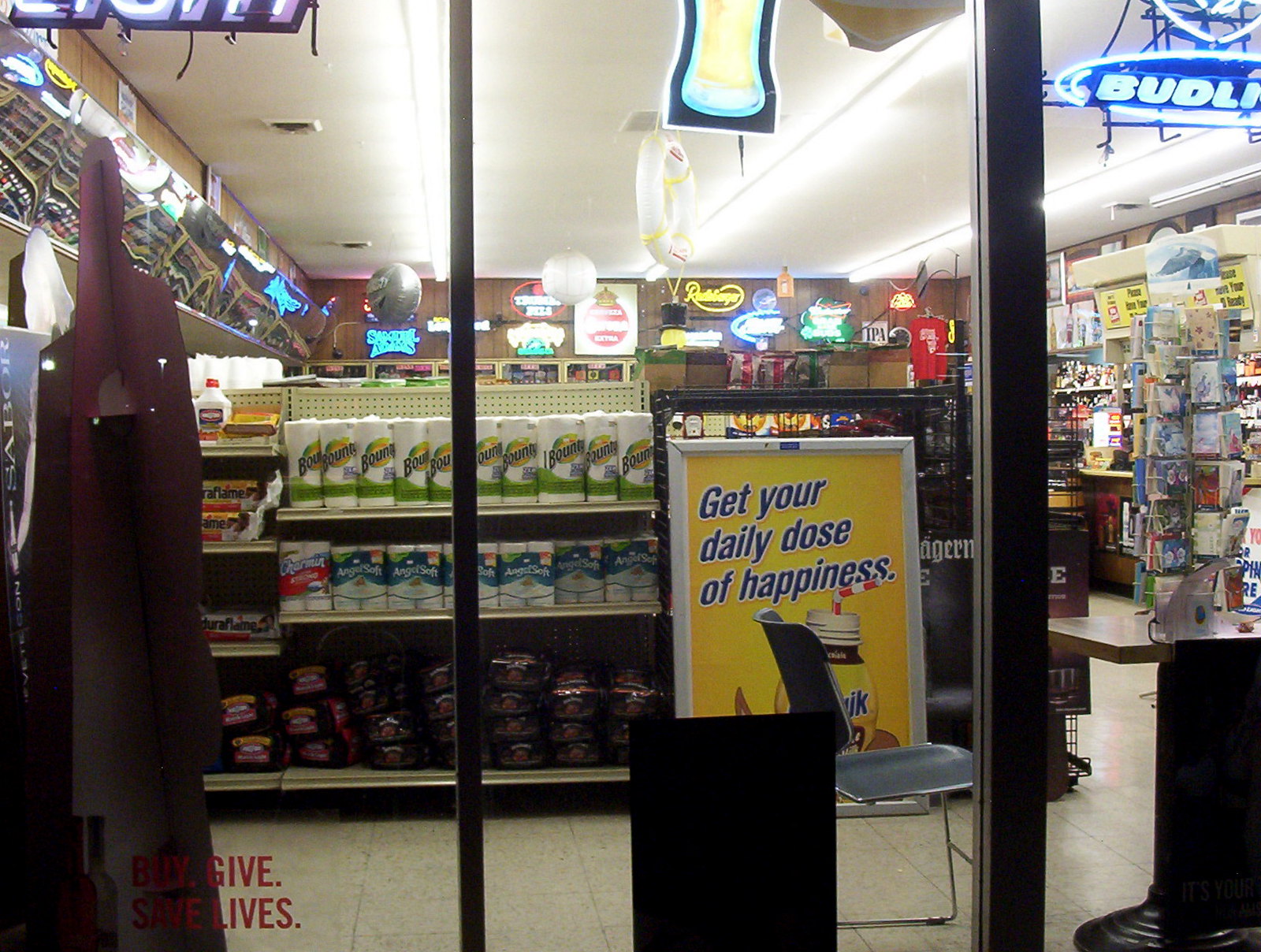This large square picture is taken outside of a convenience store, looking through its tall black-framed windows. Inside, on the upper right corner of the window, a lit-up Bud Light sign is prominently displayed. In the upper left corner, another sign, likely advertising a light beer, is partially visible. Through the center window, you can see a chair and a small desk positioned to the right. Next to the chair, a sign with a yellow background and blue print reads, "Get your daily dose of happiness," promoting Nesquik. The chair slightly obstructs the view of the Nesquik bottle. 

Further into the store, aisles are lined with products, including a front aisle stocked with Bounty paper towels, Angel Soft toilet paper below, and bags of charcoal on the bottom shelf. The backdrop of the store features a brown wall adorned with more lit-up signs, most of which advertise liquor, while the ceiling is white and fitted with fluorescent lights. In addition to the product aisles, there's a rack of greeting cards, presumably for well-wishing shoppers seeking convenience and variety.